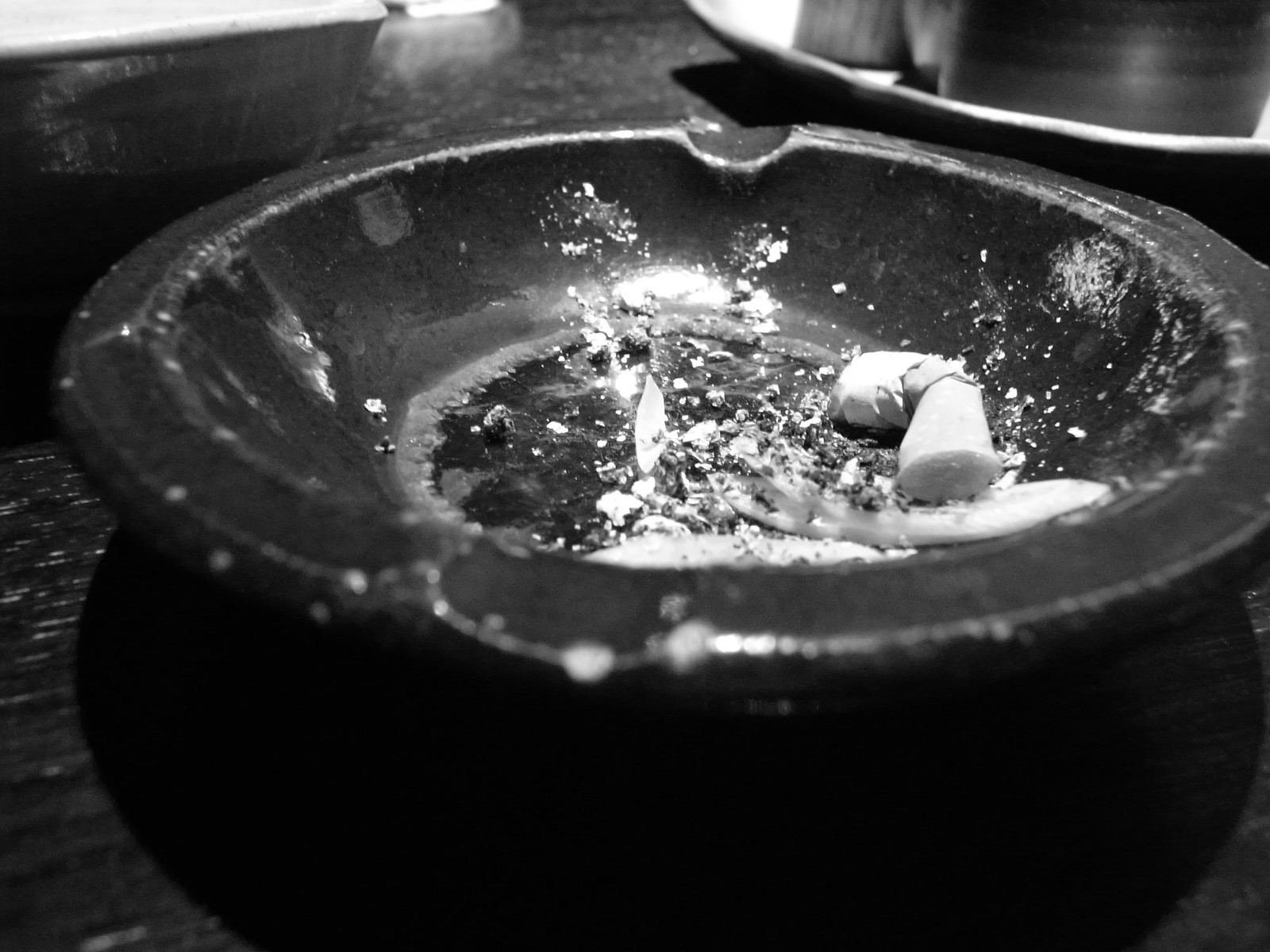This detailed black and white close-up captures a small, well-worn, black ceramic ashtray resting on what appears to be a wooden or laminate desk. The ashtray features two indentations along its edge for resting cigarettes. Within the ashtray lies a single, crumpled cigarette butt, bent to a 90-degree angle, indicating that it has been heavily smoked. The bottom of the ashtray contains a mix of black and white ashes, suggesting the cigarette was fully extinguished. The ashtray displays signs of age and frequent use, visible through chips and scratches on its surface. While the exact environment is unclear, the setting hints at a bar or diner, with indistinguishable objects—potentially other ceramic items—partially visible and cropped out of the frame.